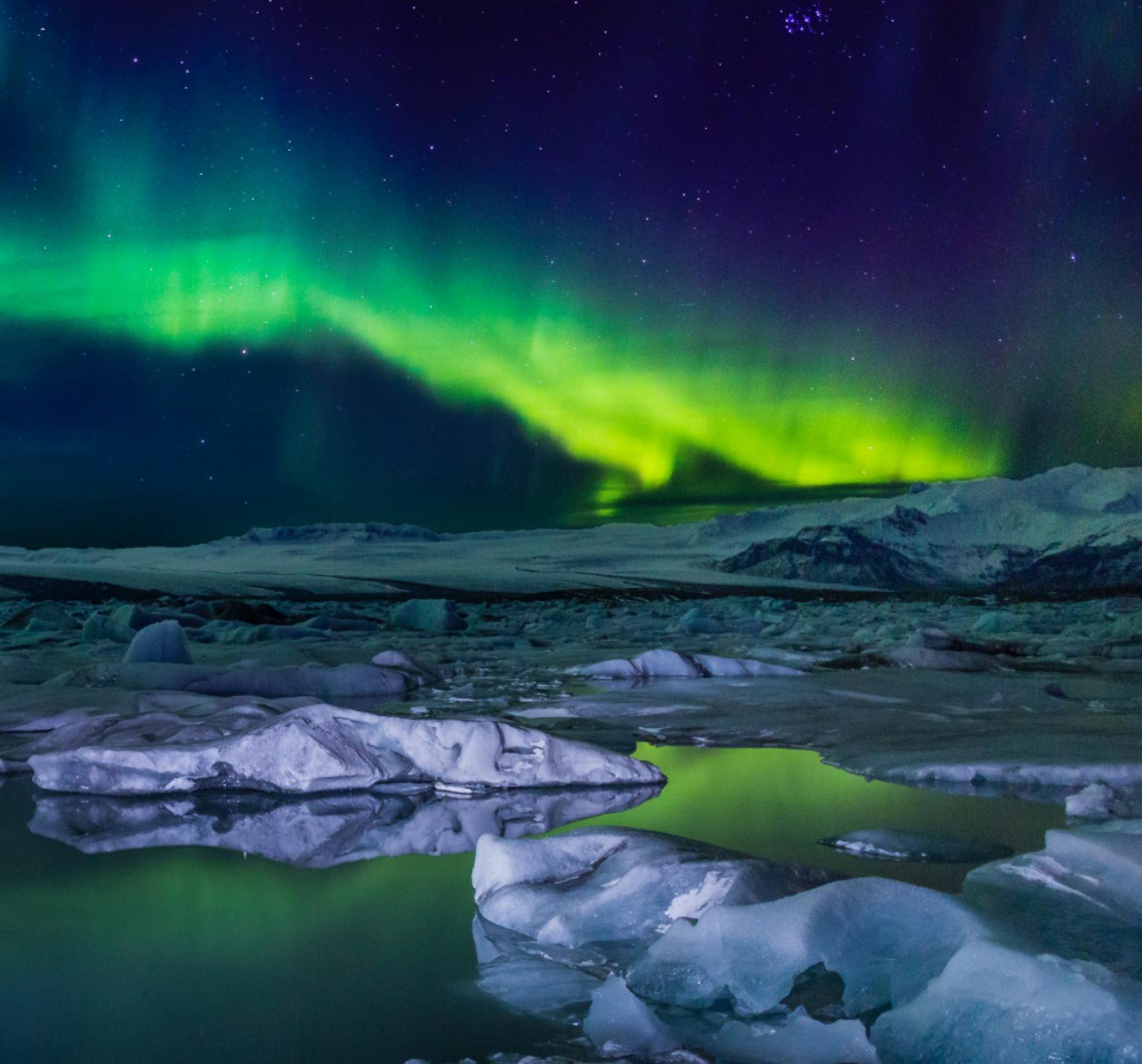The image is a square photograph of a vibrant nighttime scene, likely digitally enhanced or created. The sky, a rich indigo with hints of purple is filled with stars, predominantly in the upper right corner. Dominating the view, the Aurora Borealis displays a stunning green and yellow glow, starting from the upper left and cascading towards the center right. Below the northern lights, you find a vertical stretch of dark gray rocky terrain, giving way to a body of water where floating ice flows reflect the ethereal light from the sky. The ice contrasts with the darkness, appearing brighter amidst the surrounding reflections. The overall effect suggests a scene out of a science fiction movie, with its exaggerated colors and surreal atmosphere creating an otherworldly experience.